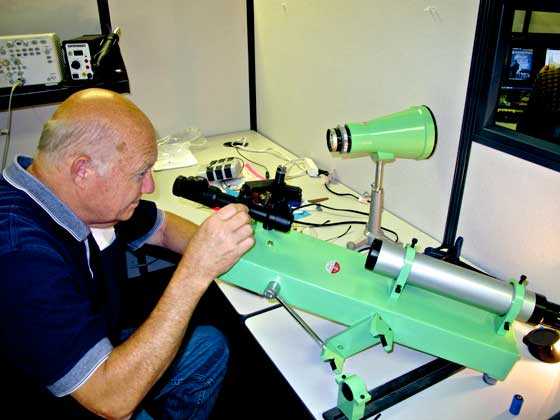In the image, an elderly man, appearing to be in his late 50s to 80s, is meticulously working at his workspace situated in what looks like an office cubicle or a laboratory. The man, who has a bald head with a touch of gray hair, is dressed in a blue polo shirt and blue jeans. He is peering intently through the eyepiece of a large, unique green instrument, which could be a microscope or a telescope, resting on a white-topped table.

The instrument itself is distinctive, featuring a mint-green cylindrical body with a black viewing tube. It is mounted on a silver stand, and an additional megaphone-like mint-green component points forward. Alongside the main instrument, a variety of smaller tools and wires are scattered across the desk, indicating a workspace filled with scientific apparatus.

To the left of the man, there's another rectangular green object, possibly a radio, contributing to the cluttered yet technical atmosphere of the environment. The office walls are white with black edges, adding to the professional yet utilitarian feel of the space.